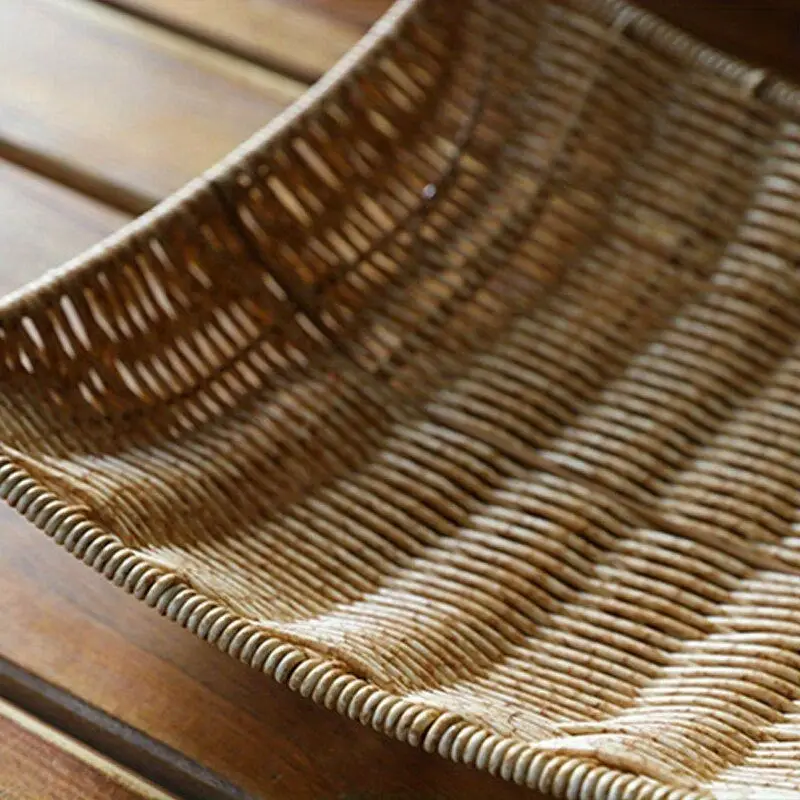The image features a wicker dish-style basket sitting on a wood table. The basket, made from thin bamboo-like reeds, has a distinctive square shape with edges that fold upwards and an inside that is somewhat rounded. Its weaving pattern is in a uniform direction, with the weft clearly visible. The basket is a light brown color with hints of browny orange, giving it subtle depth. It is about five to ten centimeters deep and lacks any handles, resembling more of a decorative bowl, potentially for holding items like fruit. The wooden table beneath it consists of multiple side-by-side slats, each approximately three inches wide, and is just a bit darker than the basket, helping the basket stand out. The image seems to capture the entire basket prominently, with no text or additional objects in view.